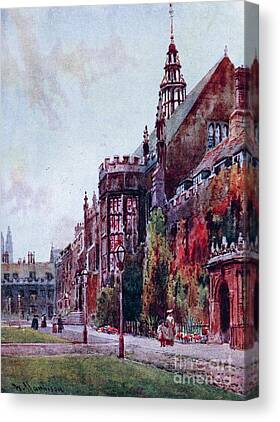This painting, created on canvas with the watermark "fine art" visible at the bottom, depicts an expressionistic portrayal of an English cityscape, likely from the early 20th century. Dominated by large, red-stone buildings featuring castle-like turrets and chapel-esque details, the scene also includes classic gas lights and red lampposts lining the street. The sky is painted with subtle clouds, suggesting a daytime setting. In the foreground, grass patches border the walkway, on which distant, indistinct figures can be seen walking, adding life and depth to the historical urban environment.